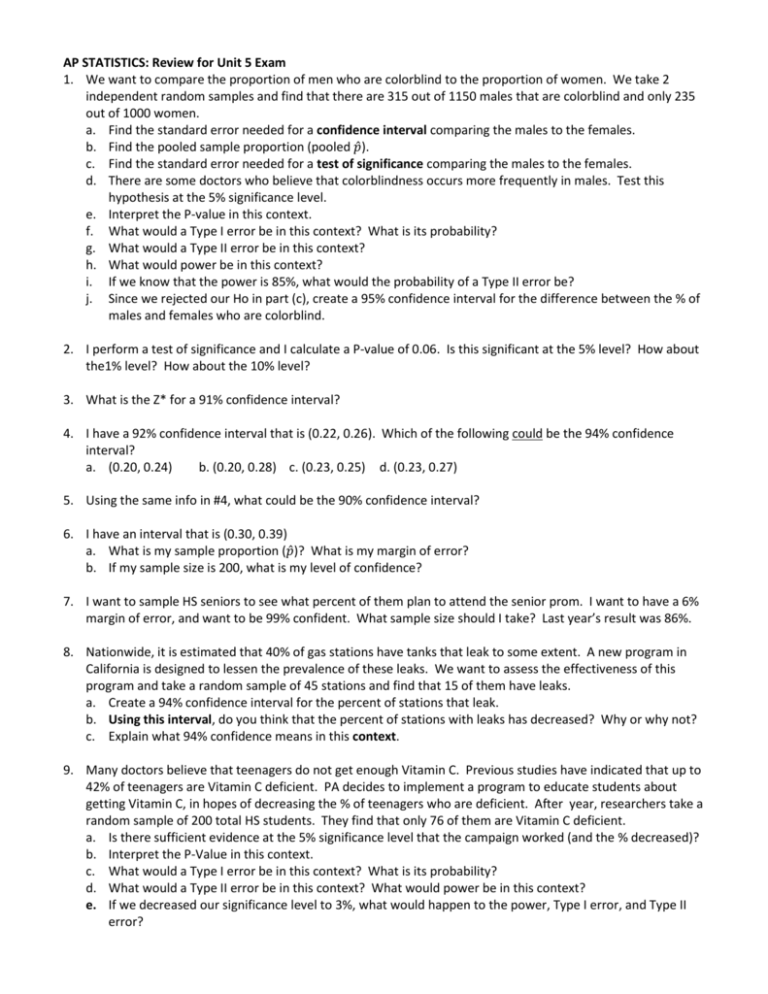**AP Statistics Review for Unit 5 Exam: Comprehensive List of Questions**

1. **Comparison of Proportions**:
   - We want to compare the proportion of men who are colorblind to the proportion of women. 
   - Two independent random samples reveal:
     - 315 out of 1,150 males are colorblind.
     - 235 out of 1,000 females are colorblind.

2. **Test of Significance**:
   - Perform a test of significance and calculate a P-value of 0.06.
   - Questions to consider:
     - Is this significant at the 5% level?
     - Is this significant at the 1% level?
     - Is this significant at the 10% level?

3. **Z-Score for Confidence Interval**:
   - What is the Z-star value for a 91% confidence interval?

4. **94% Confidence Interval**:
   - Given a 92% confidence interval of 0.22 to 0.26, determine which of the following options could represent the 94% confidence interval:
     - List of four possible answers.

5. **90% Confidence Interval**:
   - Using the information from question 4, determine what the 90% confidence interval could be.

6. **Sample Proportion and Confidence Level**:
   - Given an interval of 0.30 to 0.39:
     - Calculate the sample proportion.
     - Determine the margin of error.
     - With a sample size of 200, determine the level of confidence.

The rest of the list continues with more questions of a similar nature, focusing on error margins and statistical calculations.